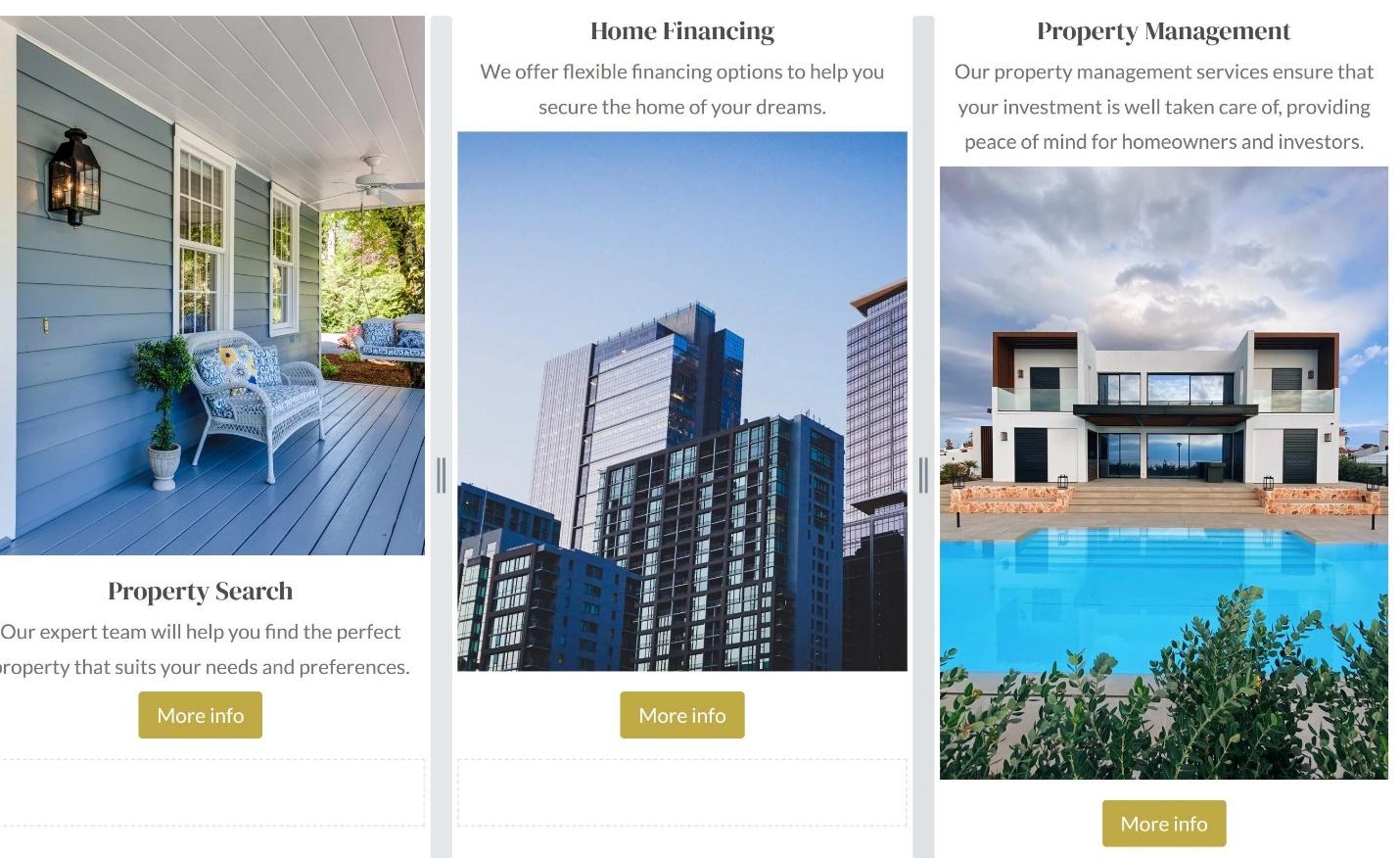This image features a collage of three distinct properties, each accompanied by text and call-to-action buttons.

**Left Image:** This is a serene photograph of a cozy, single-family home porch painted in a soothing blue hue. The porch is adorned with an outdoor sofa, a planter, and a lush green plant, while a ceiling fan provides a gentle breeze under the covered roof. The yard is a verdant oasis, brimming with greenery, and a charming lantern is mounted on the wall. Below the image, the text reads, "Property Search: Our property team will help you find the perfect property that suits your needs and preferences," accompanied by a "More Info" button.

**Middle Image:** Showcasing a corporate property, this image depicts modern commercial buildings, indicative of either a business center or luxurious apartment complexes. The text at the top states, "Home Financing: We offer flexible financing options to help you secure the home of your dreams." At the bottom, a "More Info" button invites viewers to explore further details.

**Right Image:** This image illustrates an opulent mansion with an expansive pool, signifying an upscale residential property. The accompanying text highlights, "Property Management: Our property management services ensure that your investment is well taken care of, providing peace of mind for homeowners and investors." Like the others, this segment also features a "More Info" button for additional information.